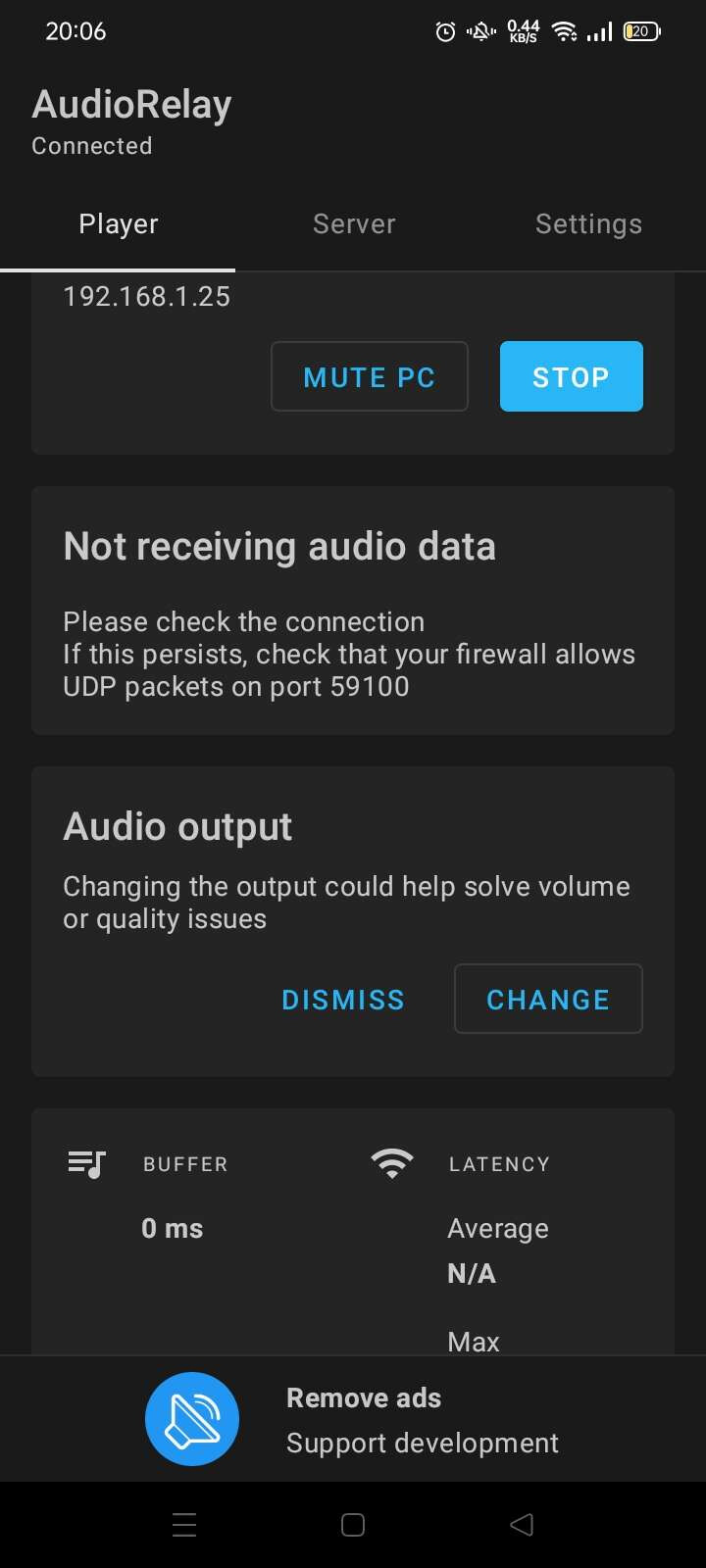The image is a screenshot from a smartphone, which appears to be in dark mode with a black background. At the top left corner, the time is displayed in white font as "20:06," using the 24-hour clock format. The top right corner shows several status icons: a nearly depleted battery at 20%, a full wireless signal strength indicated by all five bars lit up, an active Wi-Fi connection, an alarm clock icon, and a couple of other indistinct icons, one of which shows "0.44."

Beneath the status bar, on the left side, in light gray font, it reads "AudioRelay" (capitalized as one word). Below that, it says "Connected" and "Player," followed by an IP address "192.168.1.25." In the center of the screen, there are options labeled "Setting" and "Server," written spaced out. On the right side, it says "Settings."

Underneath "Setting" on the right, there is a turquoise blue rectangle with "STOP" written in white. To the left of this button, the text "Mute PC" is displayed in blue letters. Farther down is a headline in light gray font that states "Not receiving audio data." Following this, there's a message instructing the user to check the connection and, if the issue persists, ensure that the firewall allows UDP packets on port 59100.

The next section is titled "Audio Output," suggesting that charging the output could help resolve volume or quality issues. Below this, there are two blue text options: "Dismiss" on the left and "Change" on the right.

At the bottom part of the screen, a section begins with a Wi-Fi symbol next to the text "Latency." Below this, it says "Average" followed by "N/A" and then "Max." At the very bottom left, there's a blue circle with a schematic drawing that resembles a speaker. To the right of this icon, in gray font, there are two lines of text: "Remove Ads" and "Support Development."